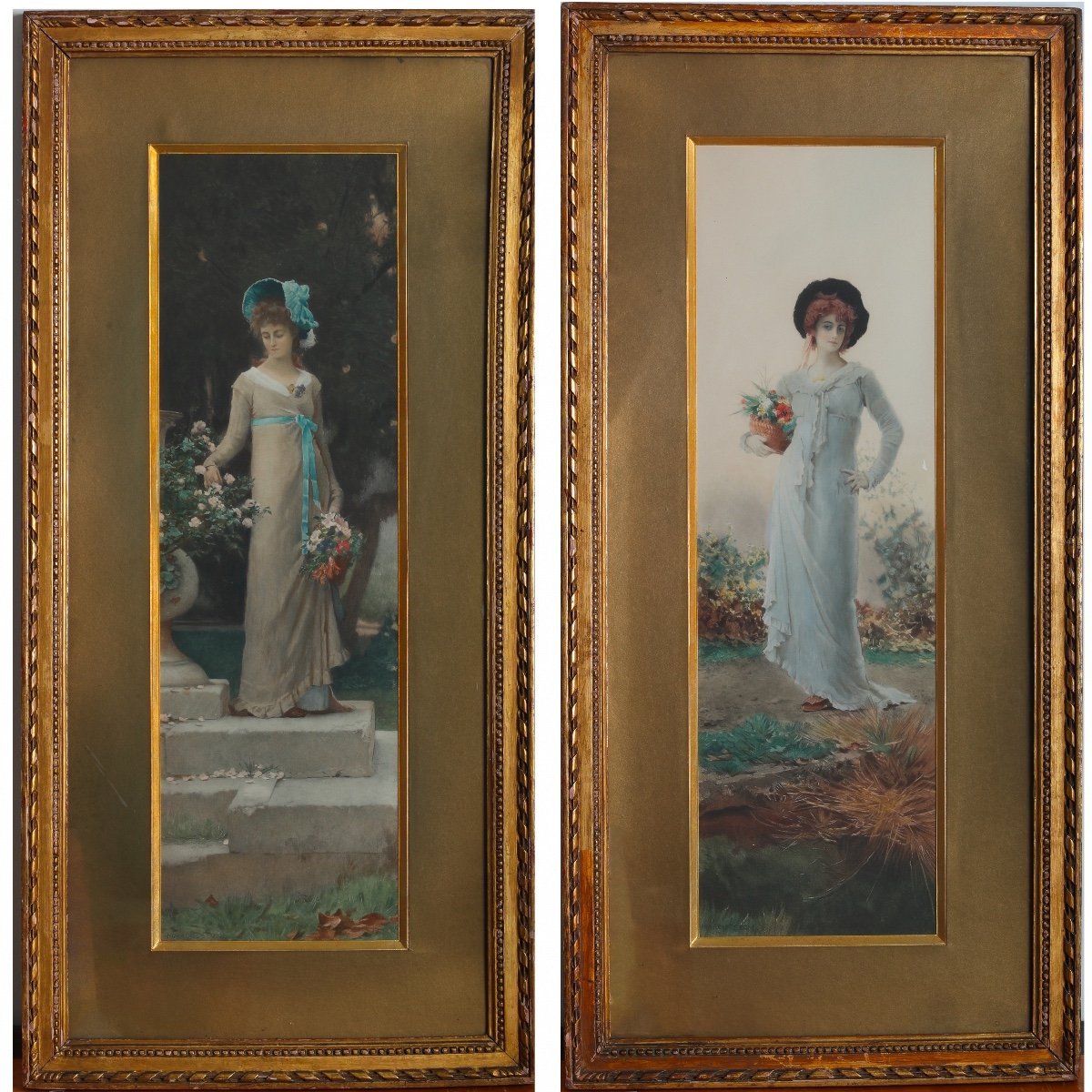The image depicts two Victorian-style paintings, framed in ornate, gold-colored frames with a gold paper border, set side-by-side on a wall, possibly in an art gallery. Both paintings feature women elegantly dressed in long gowns.

The painting on the left shows a woman wearing a beige-tan dress accented with a blue bonnet and ribbon, holding a bouquet of flowers in her hand. She stands on a set of steps next to a flower arrangement. The colors in this painting include light blue, goldish brass, pale white, beige, and reddish-brown.

The painting on the right features a woman in a white dress, adorned with a black hat, standing in a field, holding a basket filled with flowers. These paintings emphasize the detailed Victorian attire and the floral elements each woman interacts with.